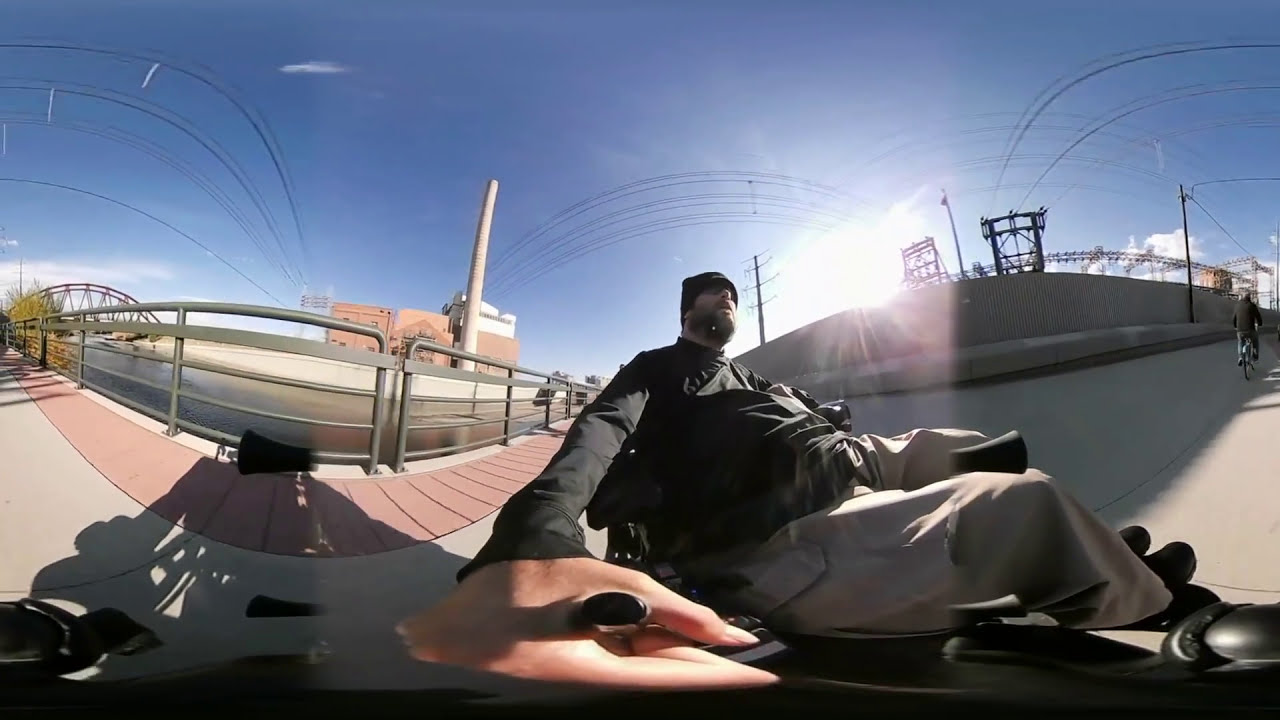The image showcases a 360-degree shot taken with a GoPro, featuring a man sitting down, likely on a bicycle, scooter, or possibly a wheelchair. He is dressed in a black coat, has a white beanie on, and light brown trousers. The man, who has a beard, is centrally positioned in the image. His right hand is prominently holding a black pole, possibly the GoPro stick or handle, which appears larger due to the perspective.

He is seated on a paved sidewalk with a brick trim, adjacent to a light gray metal railing that curves forward and back. A cyclist in a black coat is seen in the far right corner. The backdrop includes complex scenery: electrical poles and wires, a river or canal with a bridge over it, and a large factory or power station. The blue sky and sun positioned center-right add a natural contrast to the industrial elements. In the distance, possibly on the opposite side of the river, a stadium or concert venue can be seen.